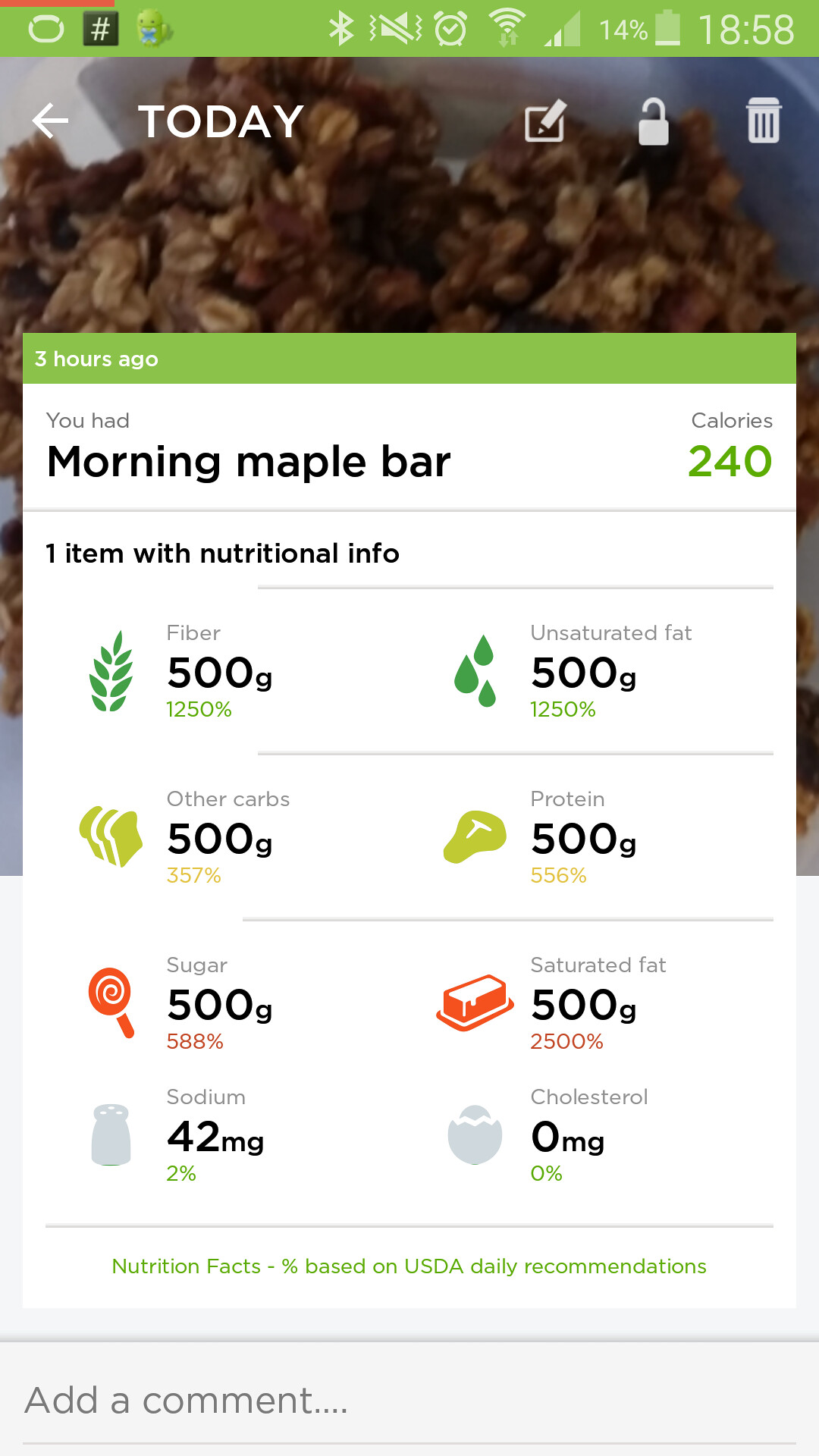The image is a screenshot of a nutritional tracking mobile application, likely taken on an Android device, given the visible status bar at the top showing a green background with various icons, a time of 18:58, and a battery level at 14%. In the upper-left corner of the screen is a small red bar, and an arrow labeled "Today" points to the left, indicating the current date. The background features an image of food, possibly a maple bar.

The screen displays a detailed report of a food entry from three hours ago, noting that the user consumed a "morning maple bar" with a caloric value of 240 calories. Below this, it lists "One item with nutritional information," followed by a breakdown of various nutritional components, each accompanied by their respective icons and values.

- Fiber: 500g, 1250%
- Unsaturated Fat: 500g, 1250%
- Other Carbs: 500g, 357%
- Protein: 500g, 556%
- Sugar: 500g, 588%
- Saturated Fat: 500g, 2500%
- Sodium: 42mg, 2%
- Cholesterol: 0mg, 0%

Each nutrient's percentage is based on USDA daily recommendations. At the bottom of the screen, there is a gray bar with an area suggesting the user can "Add a comment." The data presented is clearly exaggerated and not realistic, likely serving as a placeholder or example of how the app will function once operational.